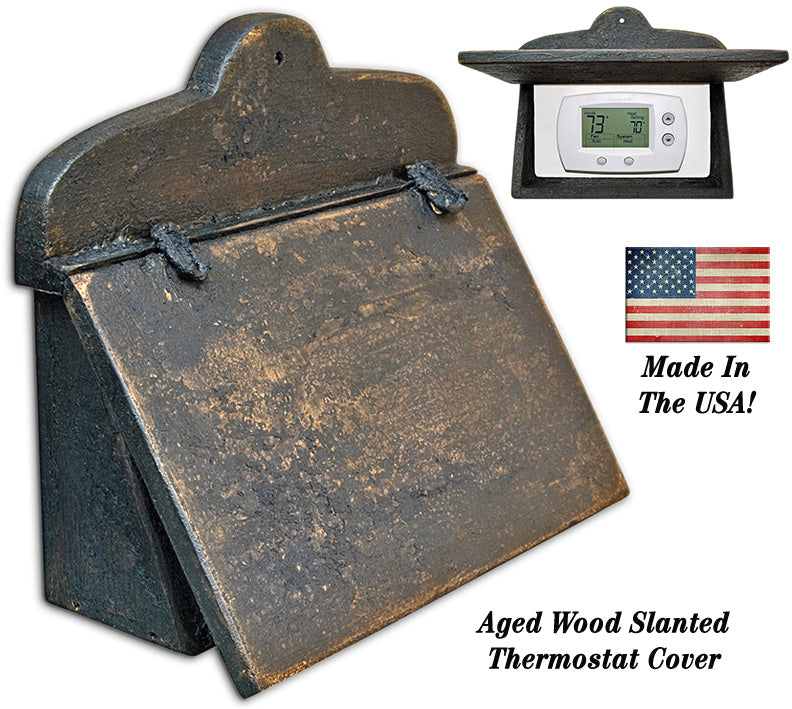This image is an ad for an "Aged Wood Slanted Thermostat Cover," set against a completely white background, giving no visible perimeter. The ad features three main components: an example photo, descriptive text, and branding elements. The centerpiece is a detailed image of the thermostat cover itself, which looks like a box with a slanted rectangular flap that can open and close to reveal the thermostat inside. The cover has a rounded top with a small hole, presumably for mounting it on a wall. The wood finish varies between dark and lighter shades of brown, giving it an antique look. Above the cover, there's an example photo showing the cover in use, open to display a white electronic thermostat reading 73 degrees. Below this, the ad includes an American flag graphic with the text "Made in the USA" in black letters, emphasizing its domestic origin. The overall design and text suggest that this is a vintage-styled item aimed at enthusiasts of aged or rustic home décor.